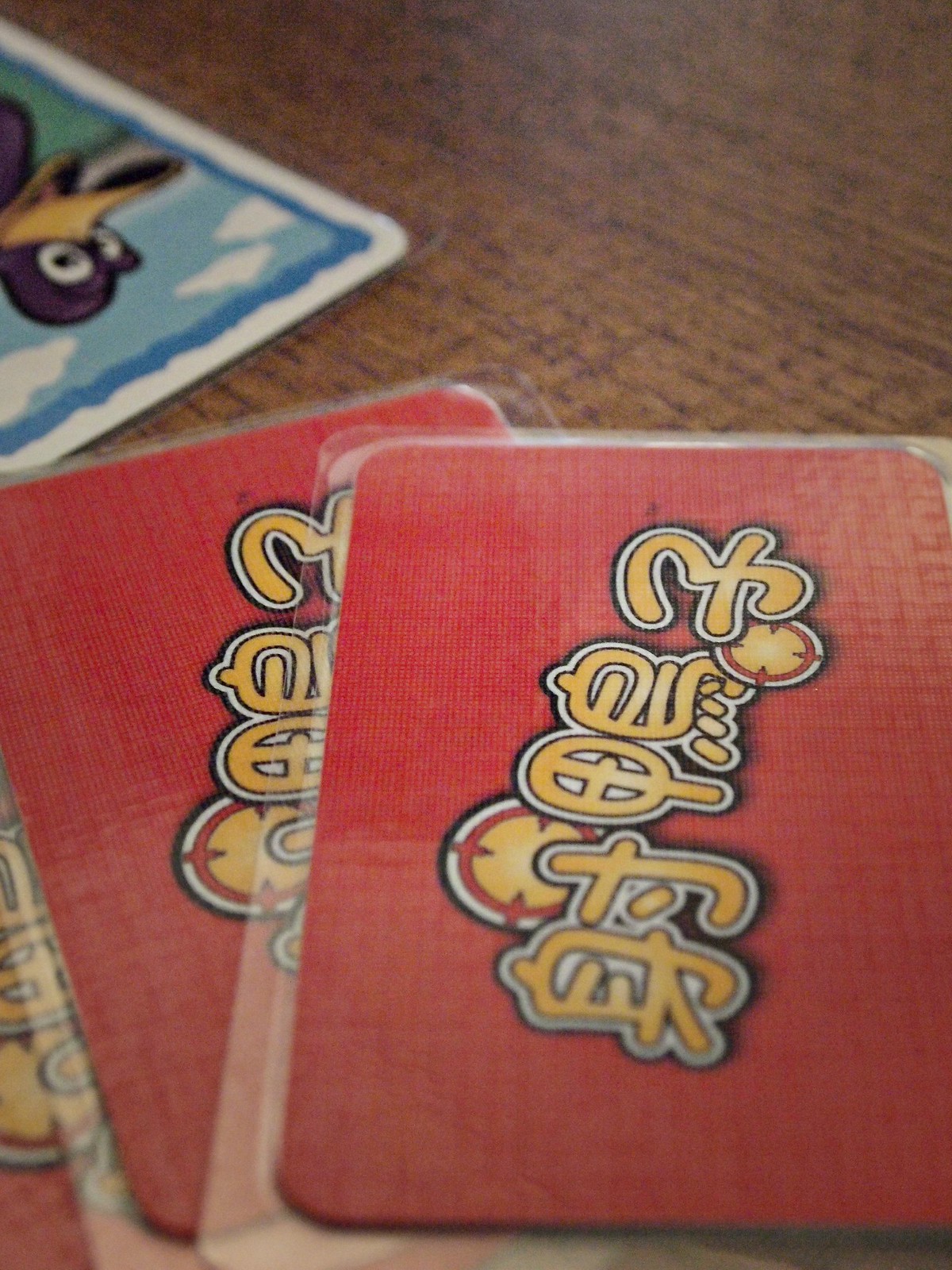This detailed photograph showcases a collection of laminated cards placed on a vintage oak table, characterized by a medium-dark stain. In the foreground, three red cards are prominently fanned out, each encased in a clear plastic laminate. The cards display striking 3D bubble lettering in a mix of yellow with a white outline, possibly featuring Chinese or another form of Asian script. Two decorative circles on each card—outlined in black and transitioning from white to red to a vibrant orange center—enhance the design, with small red dagger motifs pointing inward towards the center.

In the upper left corner, another card is notably placed face-up and upside-down. This card has a vivid, whimsical design, depicting a purple duck with a large yellow beak against a backdrop of blue sky and fluffy white clouds. The card is bordered by white and blue, adding a contrasting element to the overall scene. The artistic and colorful elements of the cards create a visually engaging composition, accentuated by the rich texture of the oak table beneath.